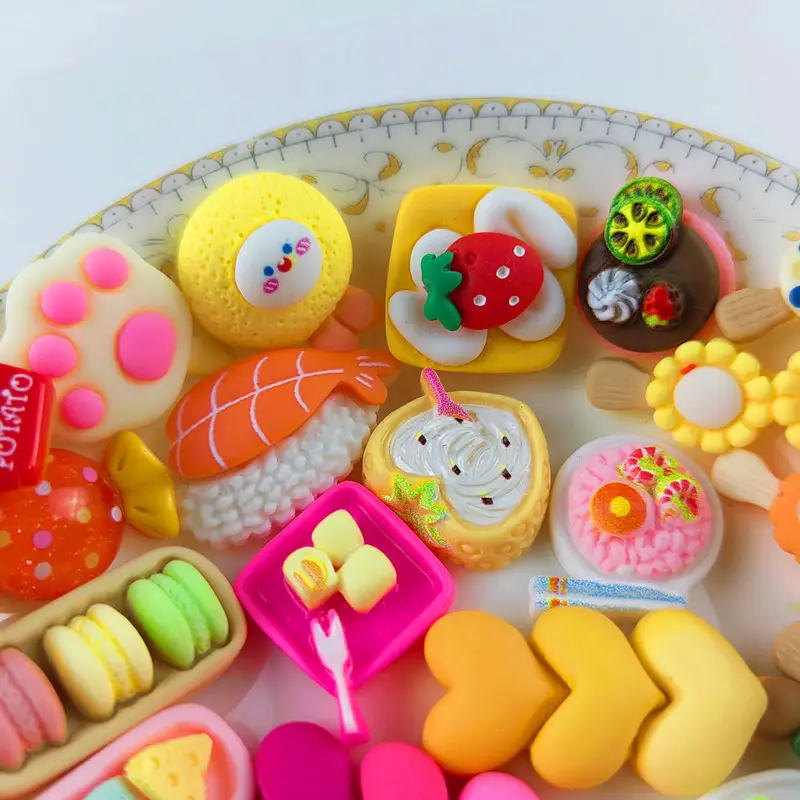The image features a white plate with a yellow border and yellow leaf designs, set against a white background. The plate is adorned with various multicolored Play-Doh creations resembling food and toys. In the lower left-hand corner, there are three vibrant green, yellow, and pink items that appear to be miniature sandwiches or cookies. Nearby, a tan paw print with five little toes sits next to a bright yellow piece with a face on it. Centrally placed is a vivid strawberry with white dots resting atop a dollop of white cream on a yellow base. There's also a pink object resembling a brain. Additionally, a yellow sunflower and three yellow heart-shaped items with some liquid inside are featured on the plate. One of the Play-Doh pieces mimics a sushi roll with rice and an orange topping that looks like salmon, complete with white fish eggs underneath.